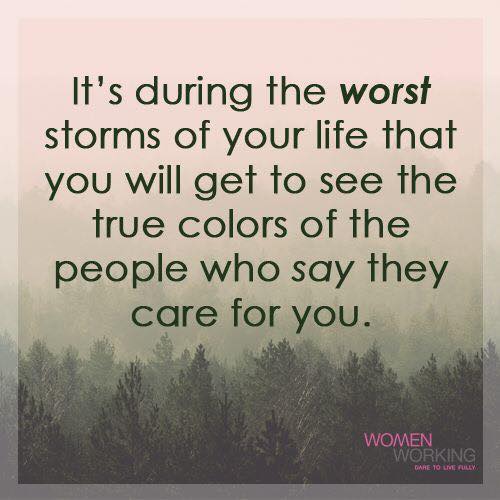The image is a motivational poster designed with a gradient overlay backdrop of foggy evergreen treetops. The upper portion of the poster features a soft reddish-pink sky, which transitions into a green-hued haze toward the bottom, providing an ethereal atmosphere. Emblazoned across the sky is a poignant message in dark forest green sans-serif font, reading: "It's during the worst storms of your life that you will get to see the true colors of the people who say they care for you." In the lower right corner, there is a logo for "women working," with "women" in bright pink and "working" in gray, followed by the slogan "dare to live fully" in all capital letters and bright pink. This graphic offers an inspirational message, ideal for social media sharing, particularly appealing to an audience seeking encouragement and support.